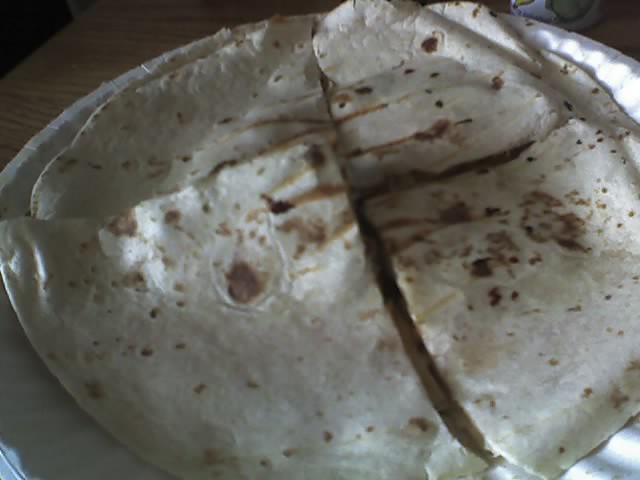A dimly lit indoor photograph showcasing a freshly baked pita bread resting on a cheap white paper plate with a fluted edge. The pita bread, which is thin yet puffy with attractive brown spots from baking, is filling most of the frame. It has been cut more or less in half, revealing its puffiness and inviting texture. The background is predominantly dark, with slight illumination around the right edge that accentuates some flutes of the paper plate. Despite the three dark corners, the pita bread stands out vividly, confirming its freshly cooked appearance.